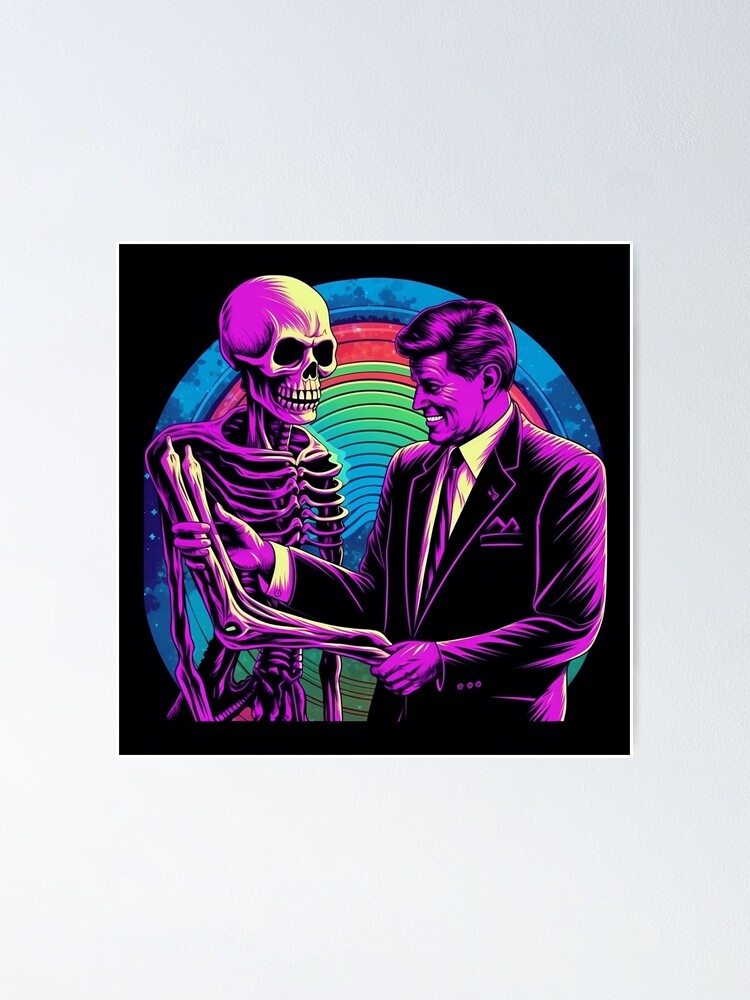This illustration depicts a man, distinctly resembling John F. Kennedy, shaking hands with a disproportionately larger skeleton, which features an oversized skull. Both figures are shaded in predominantly purple tones with highlights in white and black. The man, attired in a business suit with black, purple, and white accents, reaches out his other hand to grasp the skeleton's bicep. A wide smile is evident on both figures' faces, adding a peculiar warmth to the strange pairing. The background is adorned with a series of concentric circular rings in vibrant shades of light blue, green, and red, enhancing the surreal and AI-generated feel of the scene.